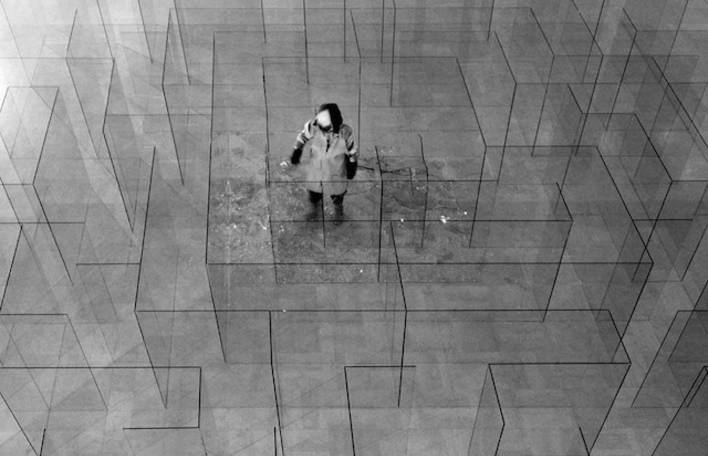In this striking black and white photograph, a lone figure stands at the center of what appears to be an intricate glass maze. The surrounding glass walls create a labyrinthine structure, with straight, reflective surfaces intersecting at various angles, creating a sense of depth and complexity. The flooring beneath the maze is tiled, with a darker central area that the individual occupies, potentially adorned with an abstract artwork. The person is clad in a long jacket that reaches their pants, paired with dark trousers and sturdy boots. Their attire is completed with long sleeves, and they have dark hair, although their features are rendered slightly blurry compared to the sharp, defined lines of the glass walls. This suggestive blurriness contrasts with the clarity of the maze, drawing attention to the enigmatic presence amidst the ordered chaos.